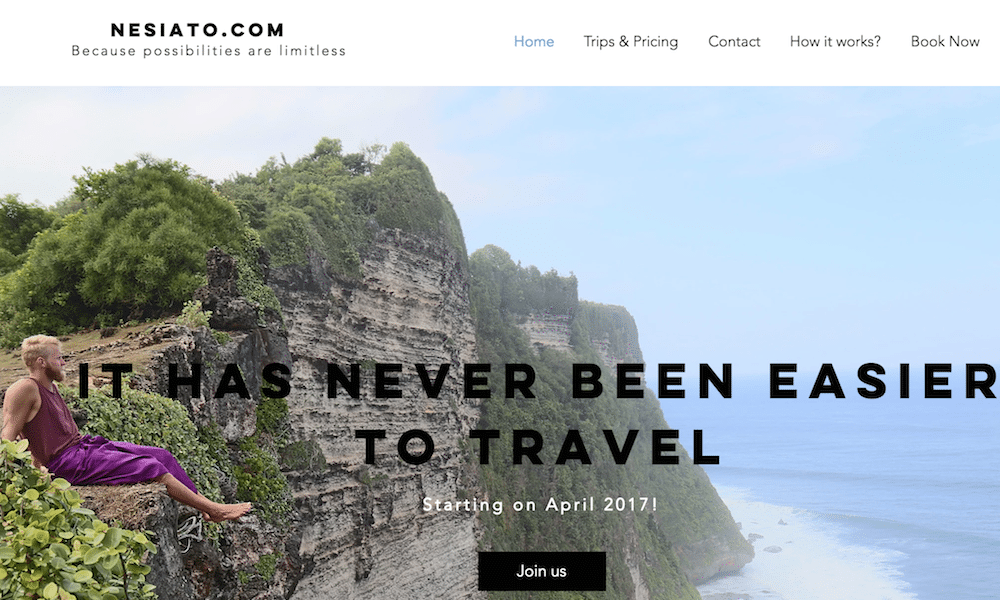The image features a clean, minimalist design with a white background and black text at the top that reads "nestiatio.com." Below this, in gray text, is the tagline, "because possibilities are limitless." In the top right corner, there is a navigation bar with "Home" in blue, and "Trips and Pricing," "Contact," "How It Works," and "Book Now!" in black.

Prominently displayed is a stunning photograph of a seaside cliff characterized by steep drops with earthy tans and browns, capped by green trees. On the left side of the cliff, a man with thick blonde hair and a brown beard is sitting, his feet dangling over the edge. He is wearing a white tank top and gazing intently at the expansive ocean below.

Overlaying the image is a bold, black text proclaiming, "It has never been easier to travel." Beneath this statement, smaller text announces, "Starting April 2017!" with an exclamation point for emphasis. Below the text, there is a conspicuous black button labeled "Join Us."

This image is part of a campaign, visually communicating the adventurous spirit and limitless possibilities offered by nestiatio.com.